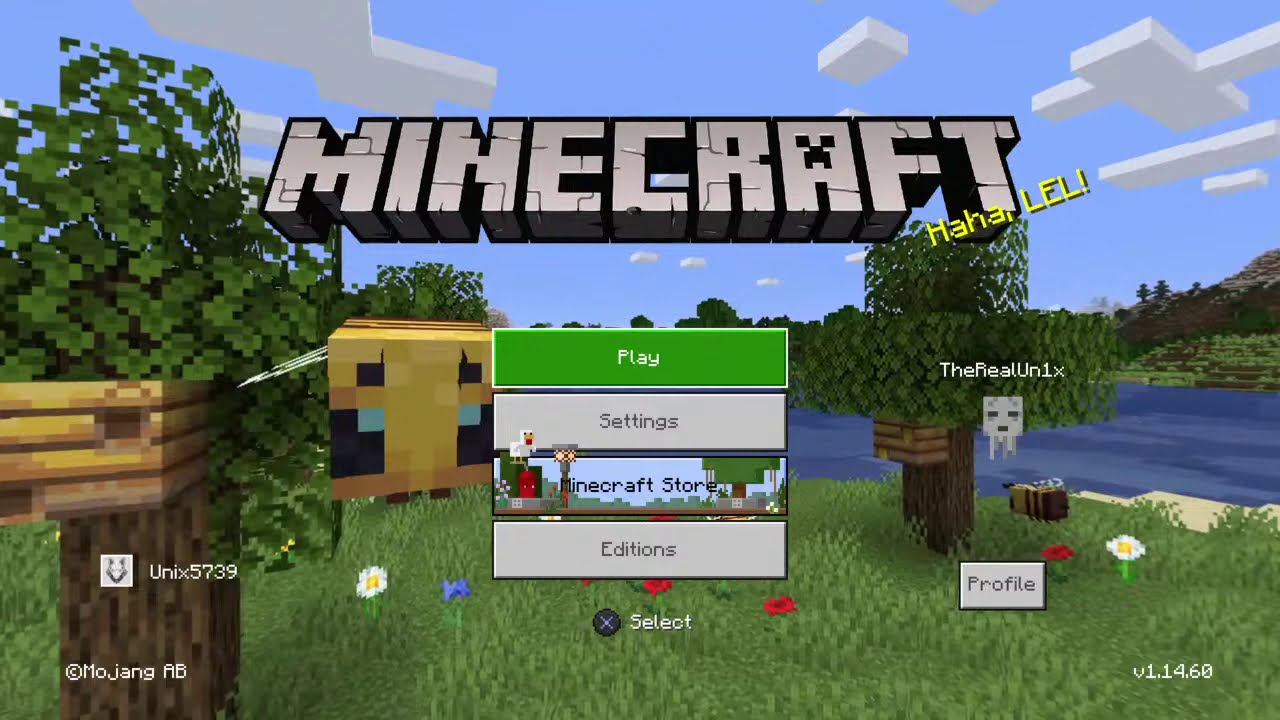The photograph captures the main loading screen of the popular video game Minecraft, depicted in a widescreen, high-definition format. At the focal point of the image, the title "Minecraft" is prominently displayed in large, white 3D block letters with a black outline, set against a vibrant backdrop featuring a blue sky dotted with cube-shaped white clouds. Below the title, there are four selectable options arranged in a vertical column: "Play" in green, followed by "Settings" in gray, "Minecraft Store" also in gray, and "Editions." 

The background image portrays a serene, computer-generated landscape with a river or stream flowing through the middle, flanked by lush bushes and trees. On the left side of the river, the foreground consists of grassy areas dotted with flowers, with more trees and some beehives visible. To the right, rolling hills and mountains add depth to the scene. An icon that reads "select" is located in the lower middle portion of the image, and various white text annotations, including a smiley face box and a username, are scattered around the edges.

The overall color palette of the screen is dominated by natural hues—blue sky, green grass, brown trees, and the blackish-gray sides of the screen—enhancing the immersive and blocky aesthetic that Minecraft is famous for.